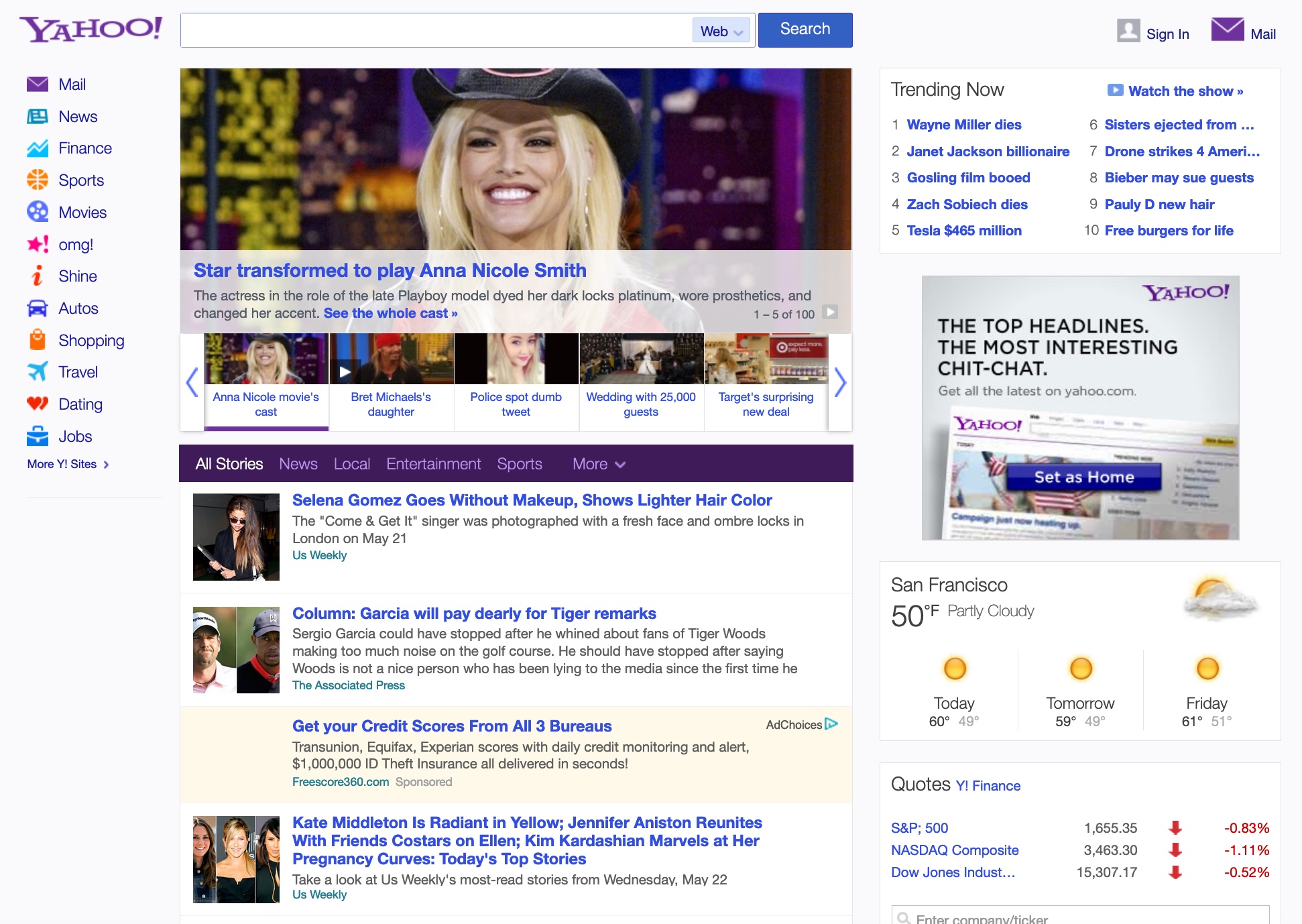Here's a refined and detailed caption for the described Yahoo main page screenshot:

---

The screenshot captures a very cluttered Yahoo main page. At the top left corner, the recognizable purple "Yahoo!" logo with an exclamation mark stands prominently. Adjacent to the logo is a search bar for web queries, accompanied by a blue search button with white text. To the left of the search bar are the "Sign In" and "Mail" buttons.

Under the logo, a horizontal navigation bar hosts a series of categories including Mail, News, Finance, Sports, Movies, OMG, Shine, Auto, Shopping, Travel, Dating, Jobs, and more Yahoo sites. Each category is marked with a distinct colored icon for easy identification.

The central area of the page features the main story titled "Star Transforms to Play Anna Nicole Smith." Directly beneath this headline is a purple bar offering more stories categorized under options such as All Stories, News, Local, Entertainment, and Sports, accessible through a dropdown menu.

Below the main story, additional news snippets are listed: "Selena Gomez Goes Without Makeup, Shows Lighter Hair Color," a column titled "Garcia Will Pay Dearly for Tiger Remarks," an advertisement urging users to "Get Your Credit Scores from All Three Bureaus," "Kate Middleton Is Radiant in Yellow," "Jennifer Aniston Reunites with Friends Co-Stars for Ellen," and "Kim Kardashian Marvels at Her 'Pregnancy Curse.'"

On the upper right side, the "Trending Now" box lists various hot topics in a compact format including "Wayne Miller Dies," "Janet Jackson Billionaire," "Ghostly in Film Mood," "Zach Sobintseff Dies," "Tesla $465 Million," "Sisters Ejected from...," "Drone Strikes," "Four Americans," "Fiber May-Sue Guests," "New Hair," and "Free Burgers for Life."

A weather widget displays the current temperature of 50°F in San Francisco, along with a forecast of highs and lows for the upcoming days. At the bottom of the page, there's a Yahoo Finance section showing the latest stock market movements.

Overall, the page is packed with information, exemplifying a very cluttered layout.

---